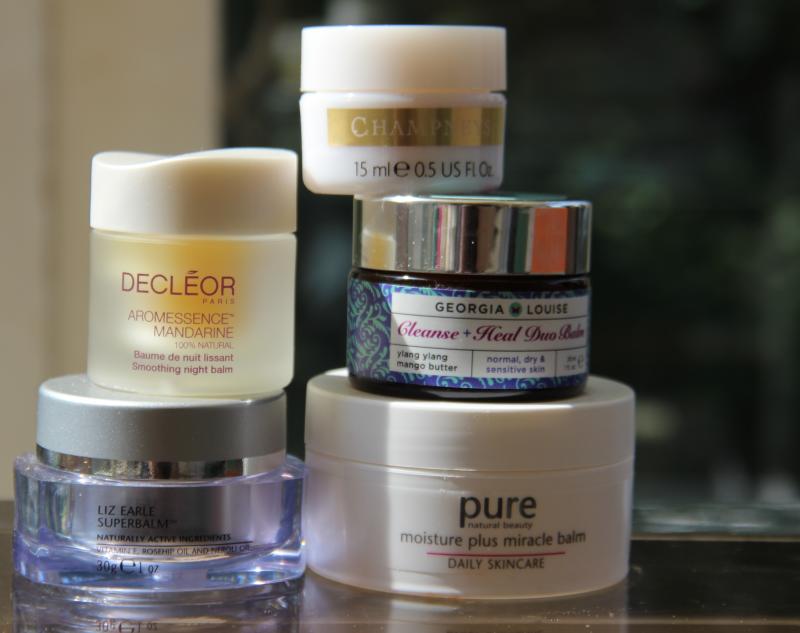The photograph features a carefully arranged pyramid of five jars of skin treatment products set against a backlit background, casting a gentle shadow in front. On the bottom left, a transparent jar with a silver lid is labeled "Liz Earle Super Balm," exhibiting a slight bluish tinge. Directly above this, a smaller jar with a white, saddle-shaped lid displays a translucent label with red and English text: "Soothing Night Balm" and references to Mandarin. 

Next to the Liz Earle jar at the bottom, there is a larger, flatter tub labeled "Pure Moisture Plus Miracle Balm Daily Skin Care," with a minimalist design. Stacked above it, a jar adorned with a paisley blue pattern and a rectangular white label reads "Georgia Louise Cleanse Heal Something Balm," where "Cleanse Heal" is written in a stylized, italic red font. 

Crowning the pyramid is a small jar with a gold label partially visible, showing the letters "C-H-A-M-P-N" and indicating a 15ml capacity. The intricate arrangement and diverse designs of the jars, highlighted by the strategic lighting, make each product distinguishable and intriguing.